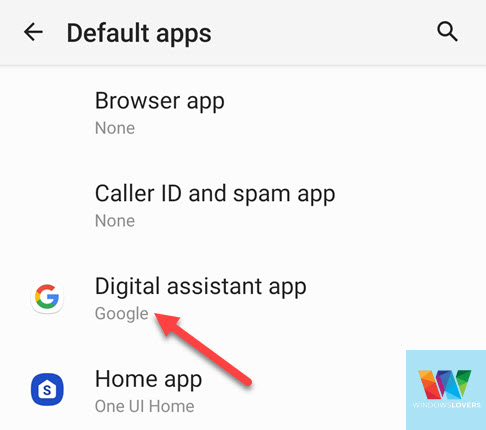This image is a detailed screenshot of a smartphone settings menu, specifically focusing on the default apps configurations. 

At the top of the screen, within a very light gray rectangle, there is a dark gray text that reads "Default apps," accompanied by a back arrow on the left and a search icon on the right. The background of the screenshot is predominantly white.

The settings options displayed are:

1. **Browser app**: Highlighted in white with the text "None" in gray beneath it.
2. **Caller ID & spam app**: Also highlighted in white, with "None" indicated in gray beneath it.
3. **Digital assistant app**: Listed with the text "Google" in gray beneath it. A red arrow is pointing to "Google," accompanied by the Google logo to the left, which is a stylized "G" comprising the colors red, yellow, green, and blue.
4. **Home app**: Displayed with "One UI Home" in gray beneath it, next to the icon for One UI Home on the left. This icon consists of a blue circle featuring a white emblem that resembles a house with a blue "S" centered within it.

In the lower right corner of the screenshot, there’s a light sky-blue square featuring an elaborate "W" logo. This logo is vibrant, incorporating a spectrum of colors including orange, red, purple, various shades of blue, and green. Beneath the "W" logo, there’s a white font text that is unfortunately unreadable. This suggests that the image is likely an advertisement utilizing a screenshot to display relevant information.